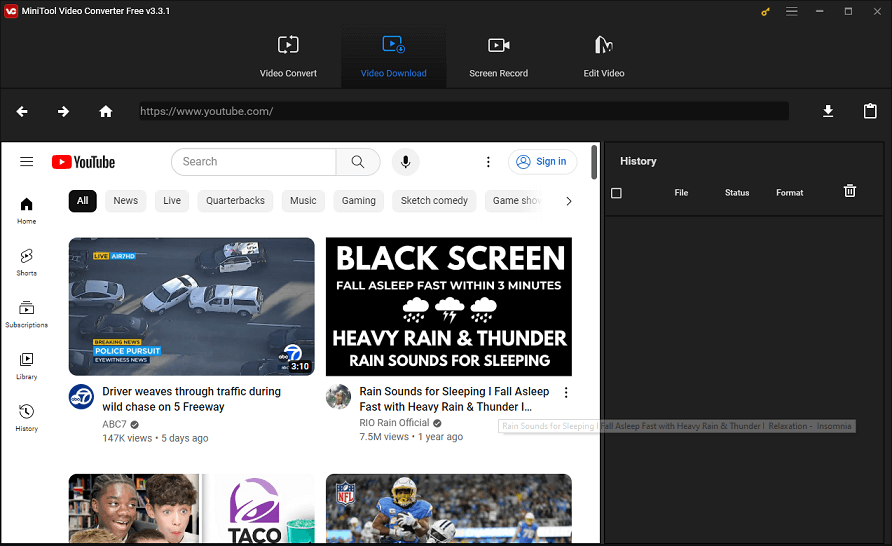A detailed screenshot of the MiniTool Video Converter Free application, version 3.3.1, is displayed on a Windows computer. The application's interface is set to dark mode, featuring a dark grey background. At the top of the interface, there are four selectable options: 'Video Convert,' 'Video Download,' 'Screen Record,' and 'Edit Video,' with 'Video Download' currently chosen.

In the 'Video Download' section, there is a field to enter a URL, with a back button, forward button, and home button for navigation. The URL 'youtube.youtube.com/' is currently entered in this field. To the right, there are download and clipboard icons for initiating downloads and copying links, respectively. 

Below this URL field, in the middle-left part of the interface, the application displays the search results for the entered URL, which is the YouTube homepage. On the right-hand side of the results, there is a history panel that shows previously downloaded videos with details such as file status and format, along with options to delete specific downloads.

Highlighted in the results is a video titled "Rain Sounds for Sleeping, Fall Asleep Fast with Heavy Rain and Thunder, Relaxation, Insomnia," indicated by the cursor hovering over it.